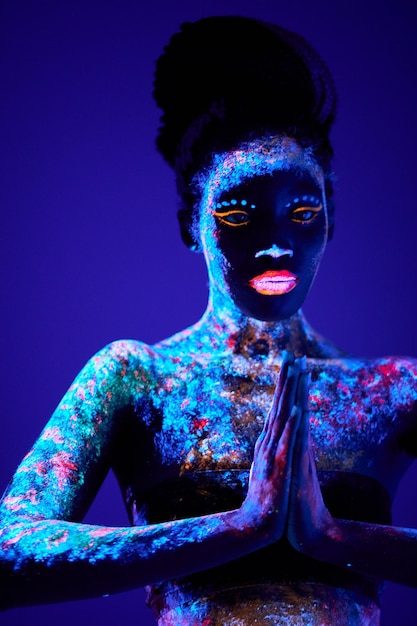The image portrays an African American woman with her hair braided and styled into an intricate updo on top of her head, set against a deep blue, almost purple background. Her face, illuminated with vibrant colors, showcases striking features: glowing pink lipstick, thick orange eyeliner encircling her eyes, and fluorescent blue dots accenting her eyebrows. The bridge of her nose is dark, but the nostrils flare with a bright blue hue. Her skin, from her face down to her chest and arms, is decorated with an array of colors, from light blues to reds, greens, and pinks, as if splattered with cosmic paint meant to glow under black light. She wears a bandeau top and positions her hands together in a praying motion, adding a spiritual or ceremonial flair to this highly stylized and artistic composition. The image is a tall portrait, slightly off-center to the right, enhancing its dynamic and otherworldly aesthetic.